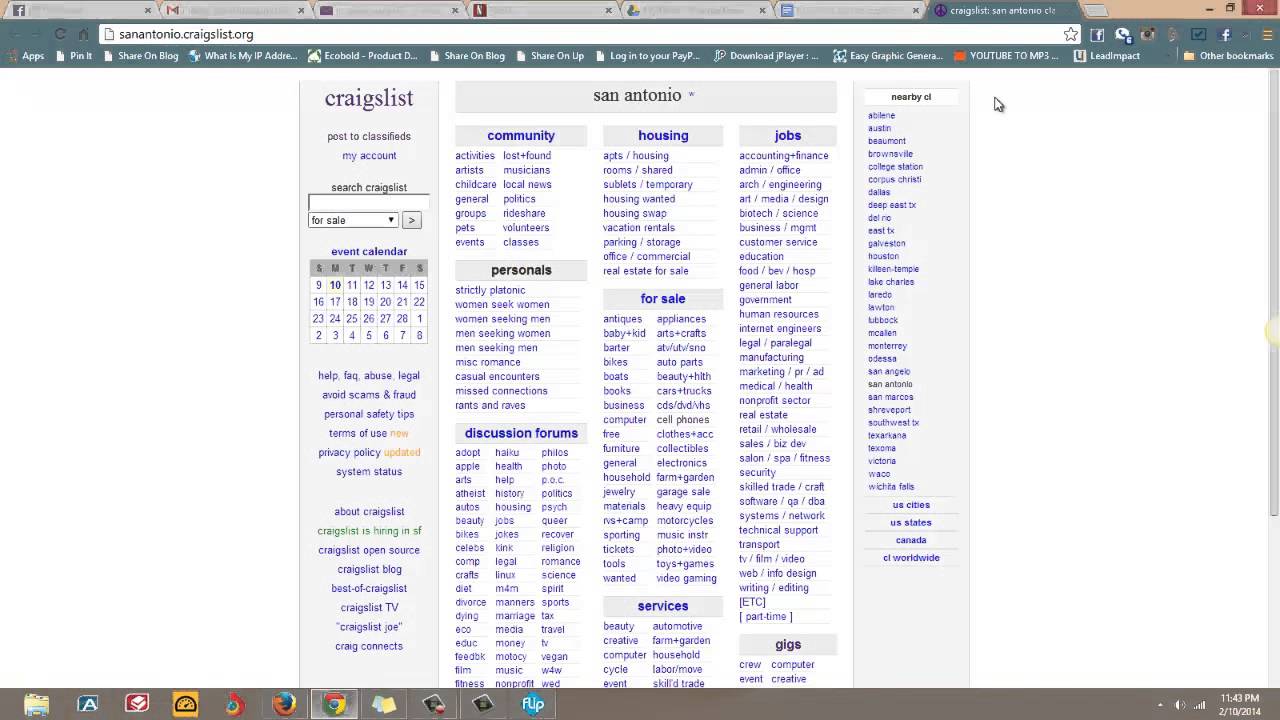The image shows a browser window with seven tabs open. The tabs include Facebook, Gmail, and the currently active tab for Craigslist in the San Antonio area. The URL bar displays "sanantonio.craigslist.org." Next to the URL bar is a star icon for bookmarking, which is currently unselected.

In the active Craigslist tab, the screen has a white background with several boxed categories linking to different sections of the website. Along the left side of the page, the words "Craigslist" are prominently displayed. Below this header, there are options to "post to classifieds," access "my account," and a search bar for navigating Craigslist listings. A calendar is visible, showing dates from Sunday to Saturday starting on the 9th and extending to the 8th of the following month.

Further down, there are links offering assistance and information about avoiding scams and fraud, FAQs, abuse and legal terms, privacy policies, system status, and general information about Craigslist. Highlighted in green, there are additional links for "Craigslist is hiring in SF," "Craigslist open source," "Craigslist blog," "best of Craigslist," "Craigslist TV," "Craigslist Joe," and "Craig Connect."

Below the general Craigslist header, specific categories are listed: community, housing, jobs, for sale, personals, discussion forums, services, and gigs. On the right side of the page, a navigation bar allows users to search Craigslist by different cities, U.S. states, Canada, and worldwide locations.